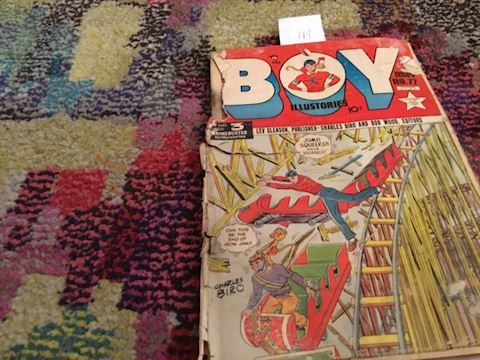A photograph captures a vintage comic book titled "Boy Illustories" resting on a vibrant, patchwork carpet commonly found in children's play areas. The carpet features a chaotic array of colors, including shades of yellow, pink, black, green, and blue. On the cover of the comic book, the title "Boy" is prominently displayed with the letter "O" containing an illustration of a boy with black hair, dressed in a red sweater and blue jeans, raising his hands to the right. Below the title, the subtitle "Illustories" is written. The cover art vividly portrays a dramatic amusement park scene, where a roller coaster is derailing, with the front car flying off the tracks. The boy in red from the title is seen clinging onto the roller coaster, seemingly leaping or attempting a rescue. A girl is seated in the front row of the derailed roller coaster, adding to the tension of the scene. There are white text boxes, possibly indicating dialogue or exclamations, while the name "Charles Byrow" is visible in the bottom left corner.